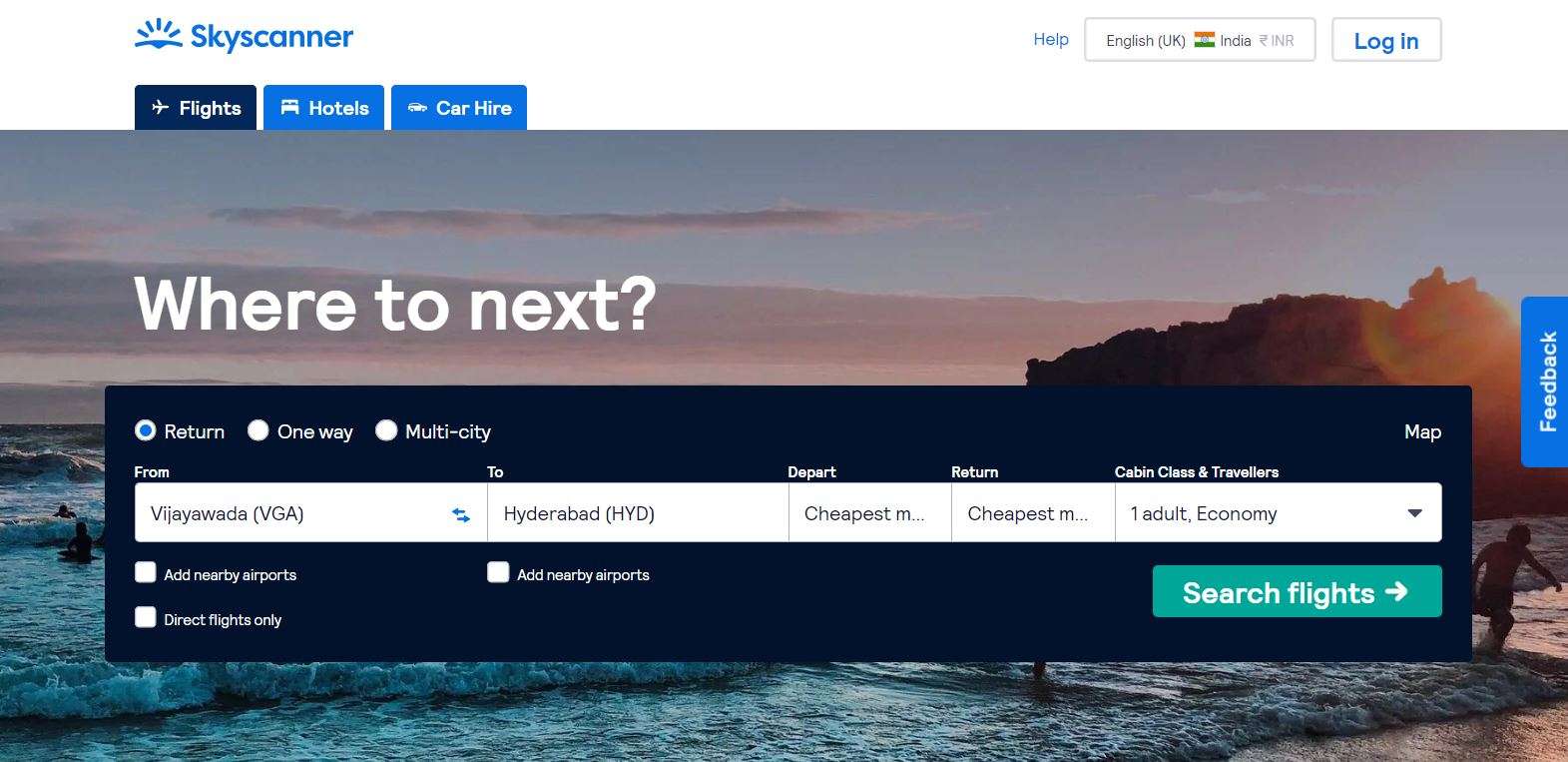The image appears to be a webpage screenshot from Skyscanner, featuring a serene and picturesque scene resembling either sunrise or sunset over the ocean. At the top of the page, there's a prominent white border with "Skyscanner" written in blue. On the right, a blue hyperlink labeled 'Help' is visible, along with a language selection box showing 'English' and the Indian flag indicating the country as India. Additionally, there's a white login button with 'Login' written in blue. 

Below the top border, there's a navigation section with three boxes labeled 'Flights,' 'Hotels,' and 'Car Hire.' The main background image features a clear blue sky with purple hues, indicative of dusk or dawn, and a tranquil ocean with gentle waves lapping at the shore. People can be seen playing by the water, enhancing the lively yet peaceful atmosphere.

Prominently placed in the center of the image is text in white letters that read "Where to next?" There is also a search box labeled with options for 'Return,' 'One Way,' and 'Multi-city' journeys, along with input fields marked 'From,' 'To,' 'Depart,' and 'Return.'